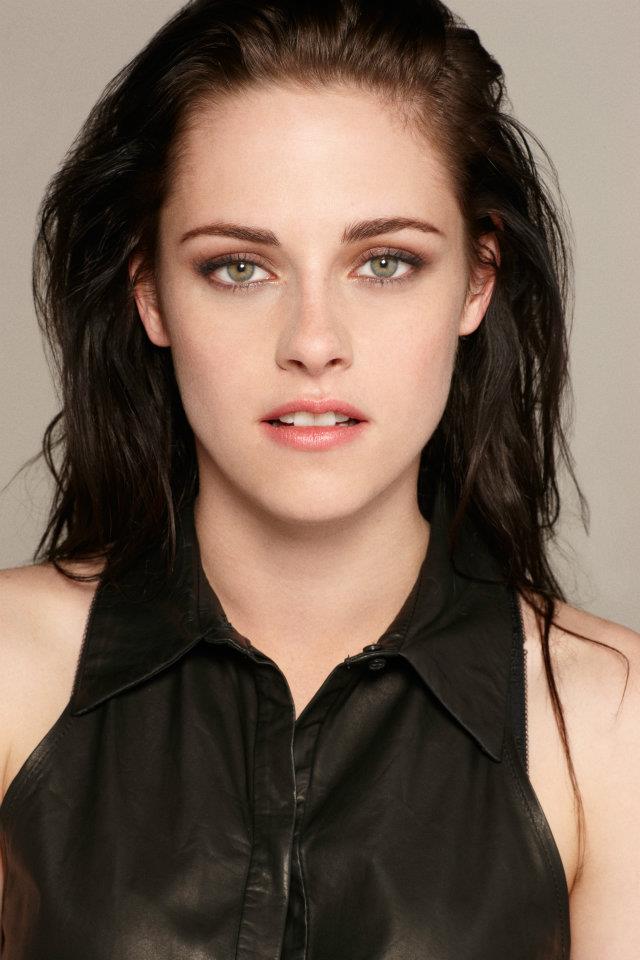The image is a detailed, close-up color photograph of actress Kristen Stewart. She appears to be in her late 20s to early 30s, looking directly into the camera with a faint, partial smile that reveals the top row of her teeth. Kristen has dark brown, tousled hair swept back, and striking greenish eyes accentuated with eye makeup. Her complexion is quite pale, and she's wearing a light red lipstick. She is dressed in a sleeveless black button-up collared shirt that possibly has a leather texture, allowing a glimpse of her bare shoulders and upper chest. The background is a plain light gray or beige wall. The top of her head is slightly cut off in the frame, emphasizing her face and upper body in a realistic, photographic style.